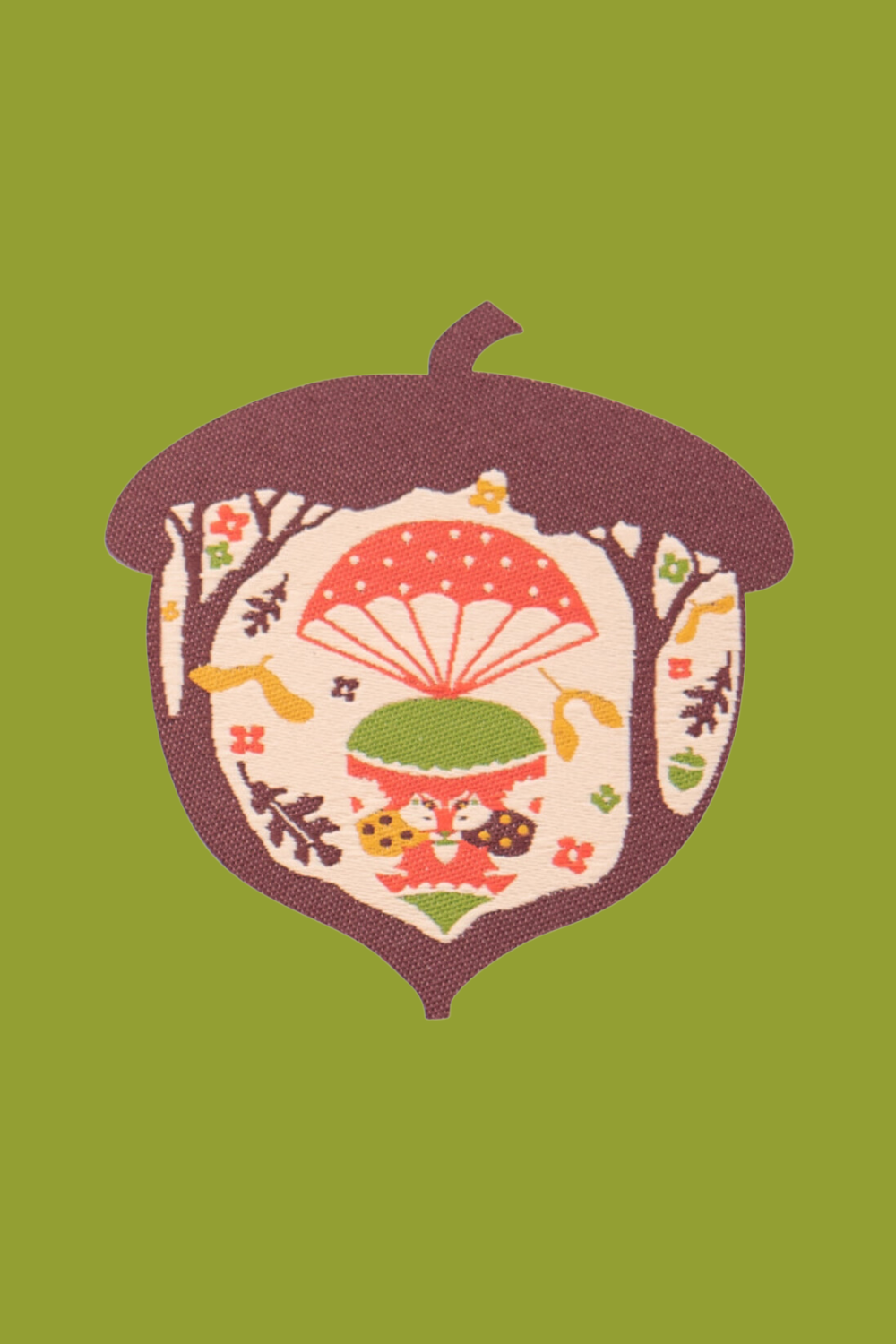The image is a detailed artistic rendering of an acorn against an avocado-green background, reminiscent of a poster. The deep brown acorn cap features a small stem protruding from its top. Intricately drawn into the acorn is a raindrop-shaped green object with various interior designs. At the top of this shape is an orange and white parachute adorned with dots. Below the parachute, within the green shape, a tiger face is set against an orange background. The acorn also contains multiple small elements such as orange and green flowers, brown and yellow leaves in various shapes, red flowers, yellow birds, smaller green acorns, and green and yellow stars. All these details come together in rich, vibrant colors, creating a complex, whimsical scene.